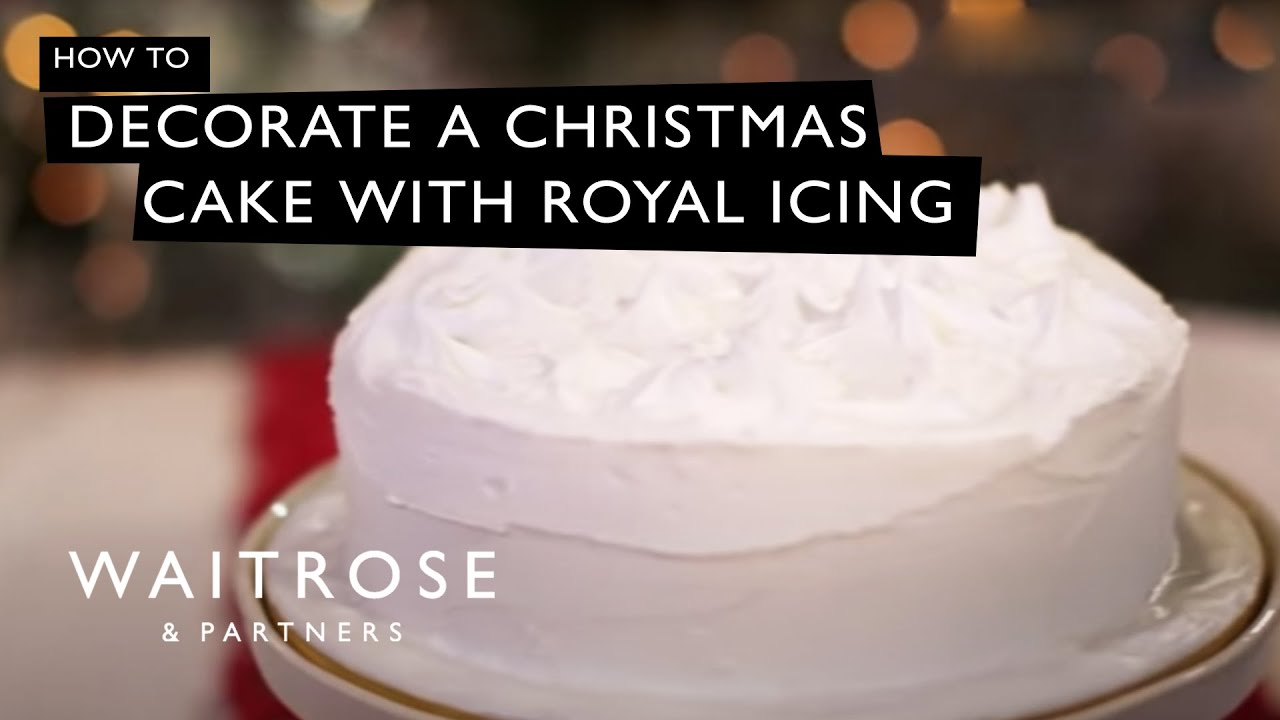This digital poster features an instructional advertisement on decorating a Christmas cake with royal icing. The focal point is a small, round, white cake with smooth white frosting, placed on a white plate with a gold rim, which itself sits atop a red runner. The cake appears slightly offset to the right, while the background is blurred, showcasing a gradient from a cream-colored lower area to a dark brown upper region, sprinkled with orange and yellowish dots.

In the top left corner, white text against a black background reads, "HOW TO DECORATE A CHRISTMAS CAKE WITH ROYAL ICING." In the bottom left corner, also in white text, it states, "WAITROSE & PARTNERS." This detailed visual invites viewers to a step-by-step guide on creating festive cake decorations, presented in a clear and visually appealing manner.